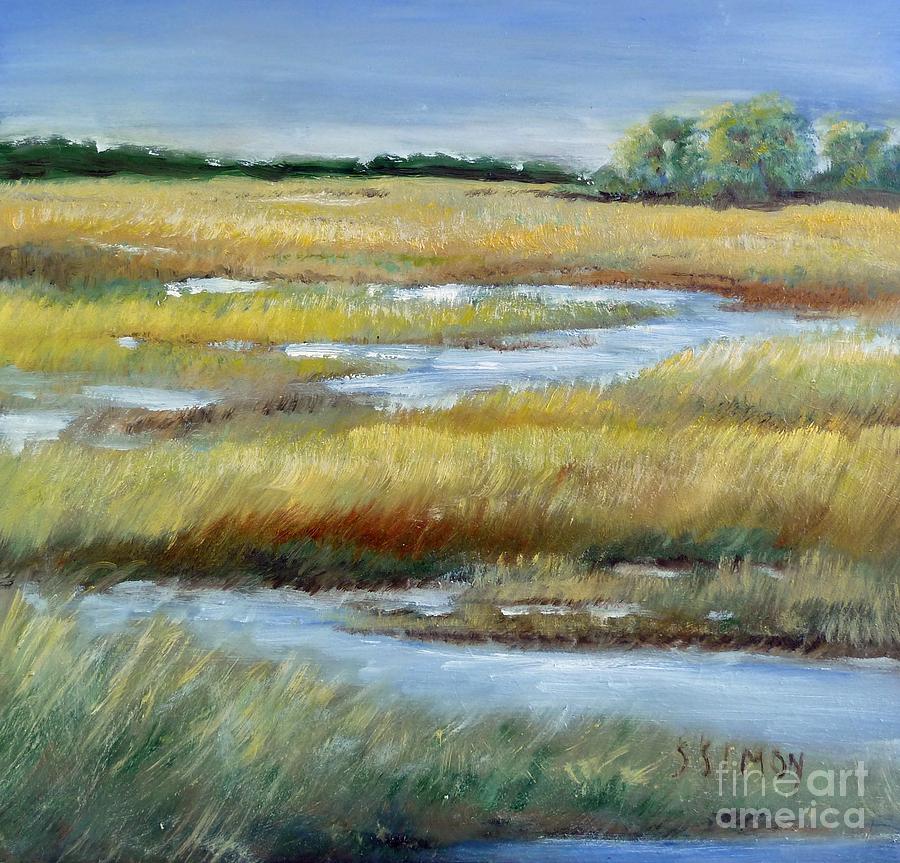The image depicts a square, impressionistic painting of marshland under a blue sky. A line of green trees and bushes forms a backdrop beneath the sky, tapering toward the distant horizon. Below this, the scene transitions into a complex, layered landscape featuring a meandering stream that snakes through the marsh. The water's surface is dotted with varying grasses, predominantly green in the foreground, shifting to yellows towards the background, suggestive of rushes or boggy growth. The grasses appear to lean slightly to the right, perhaps stirred by a gentle breeze. The detailed brushstrokes emphasize the texture and movement within the painting, which is signed “S. Simon” in the lower right corner, above a watermark indicating it's part of the Fine Art America collection.